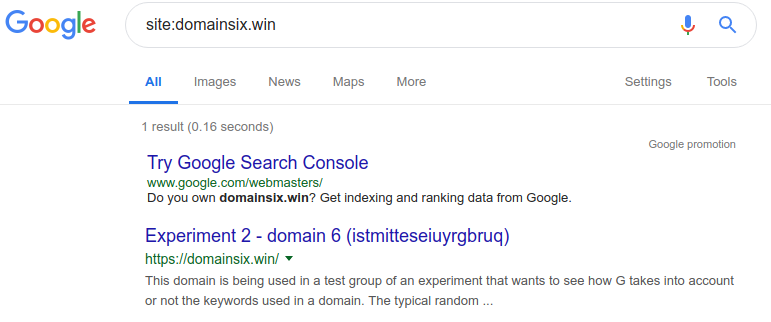The image depicts a Google search results page. In the search field, the query "site:domain6.win" is entered. To the left of the search field, the iconic Google logo appears in its traditional colors of blue, red, yellow, and green. Below the search field, there's a snippet of text promoting the use of Google Search Console, with a link: "www.google.com/webmasters/". The text also inquires if the user owns the domain "domain6.win" and suggests using the service to gather indexing and ranking data from Google.

Additionally, a highlighted search result titled "Experiment 2" refers to the domain "https://domain6.win/". This domain is part of a test group designed to investigate how Google's search algorithms account for or ignore keywords within the domain name.